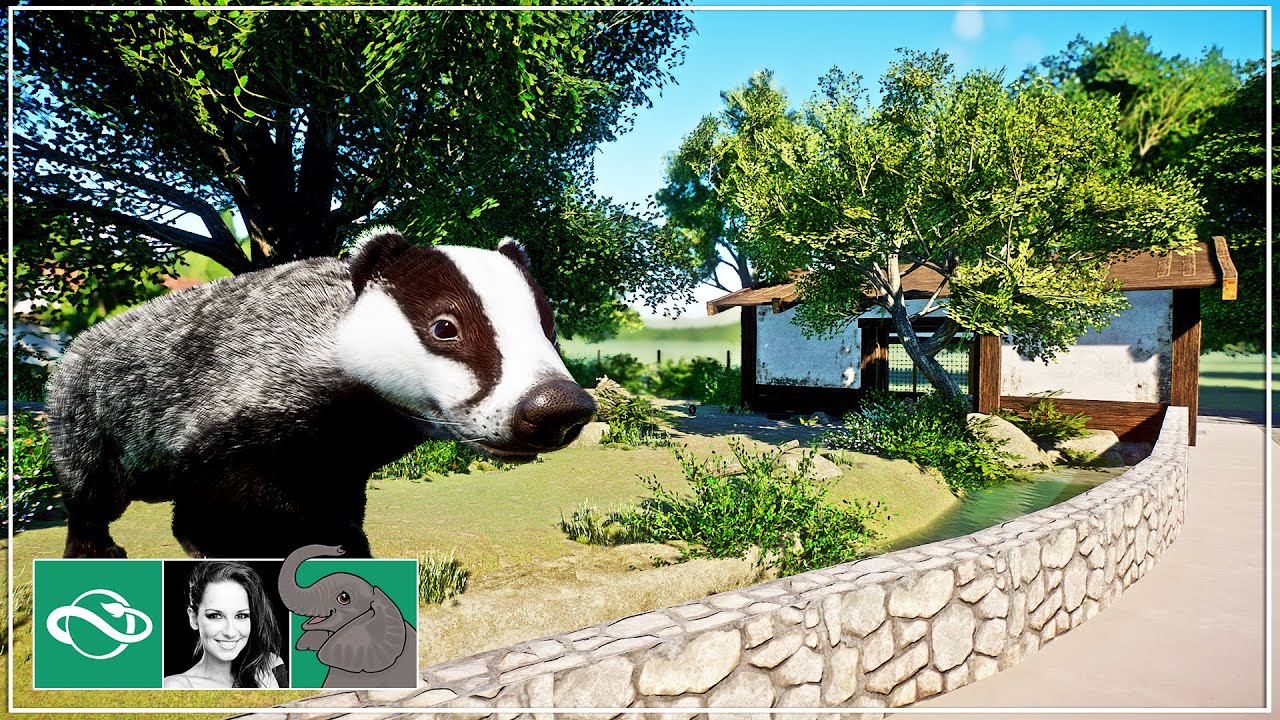This image appears to be a computer-rendered depiction of a zoo exhibit, featuring a surreal scene. Dominating the middle of the image is an oversized badger—gray, with a white and brown face—standing in a grassy, park-like area behind a round gray stone wall. The background includes a tall green tree, several smaller trees with lush green leaves, a rock barrier, and a small body of water near the wall. On the right side, there's a small white shed with a brown roof partially obscured by vegetation. The sky is blue and clear, adding to the serene ambiance. Below this scene are three small squares: the first on the left has a green background with a white circle and possibly a tail or snake symbol; the middle one contains a black and white photograph of a young brunette woman's face; and the one on the right features a drawing of a gray elephant against a green background. This highly detailed image captures the essence of a zoo exhibit with an almost animated quality.